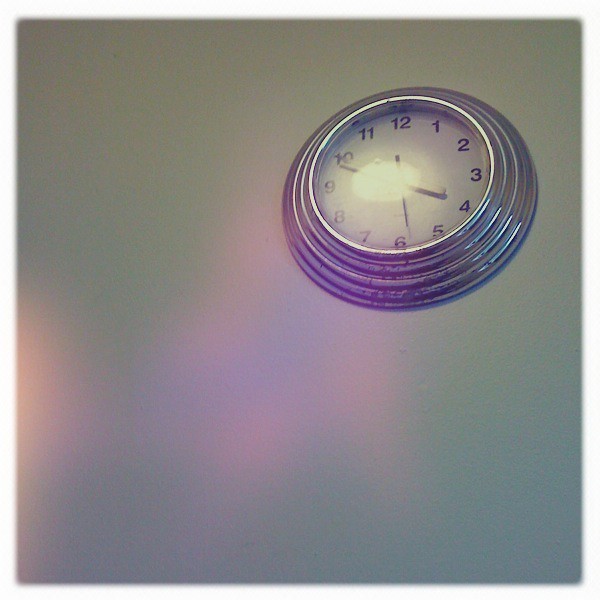This detailed photograph depicts an analog clock mounted on a white wall, specifically positioned in the upper right-hand corner of the image. The clock features a casing comprised of several concentric silver rings that enlarge as they radiate outward from the clock's face, giving it a distinctive cylindrical texture. Enclosed within a glass or plastic dome, the clock face displays standard black numbers from 1 to 12 arranged in a clockwise manner. The clock is equipped with a prominent black minute hand and a slightly shorter black hour hand, indicating the time is approximately 5:49, with some ambiguity due to the intense glare making it difficult to confirm the presence of a second hand. The photograph is taken from a low angle, emphasizing the clock's elevated position on the wall and capturing a pink light reflection that subtly tinges the otherwise white background.